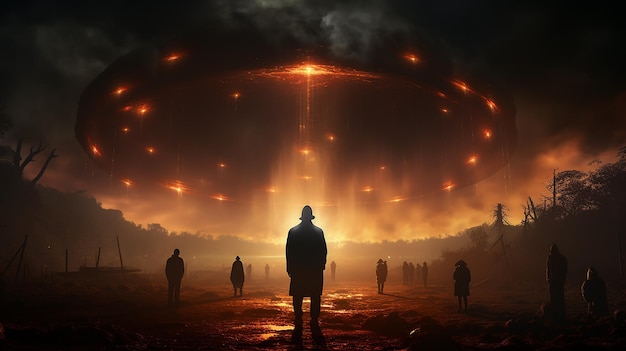In this captivating sci-fi or fantasy scene, a group of adults—both men and women—gathers in a recently rain-soaked dirt area, their reflections mirrored in scattered puddles. The backdrop features a dense, forested area, but the true spectacle lies in the sky above. Dominating the heavens is a circular object, potentially a spaceship, encircled by an array of small, glowing orange lights that highlight its rim. At the center of this celestial phenomenon, a larger, intensely bright orange light beams down, suggesting the dramatic act of someone either being transported to or from the enigmatic spacecraft. The contrast between the earthly setting and the extraordinary skyward event creates a mesmerizing and otherworldly atmosphere.